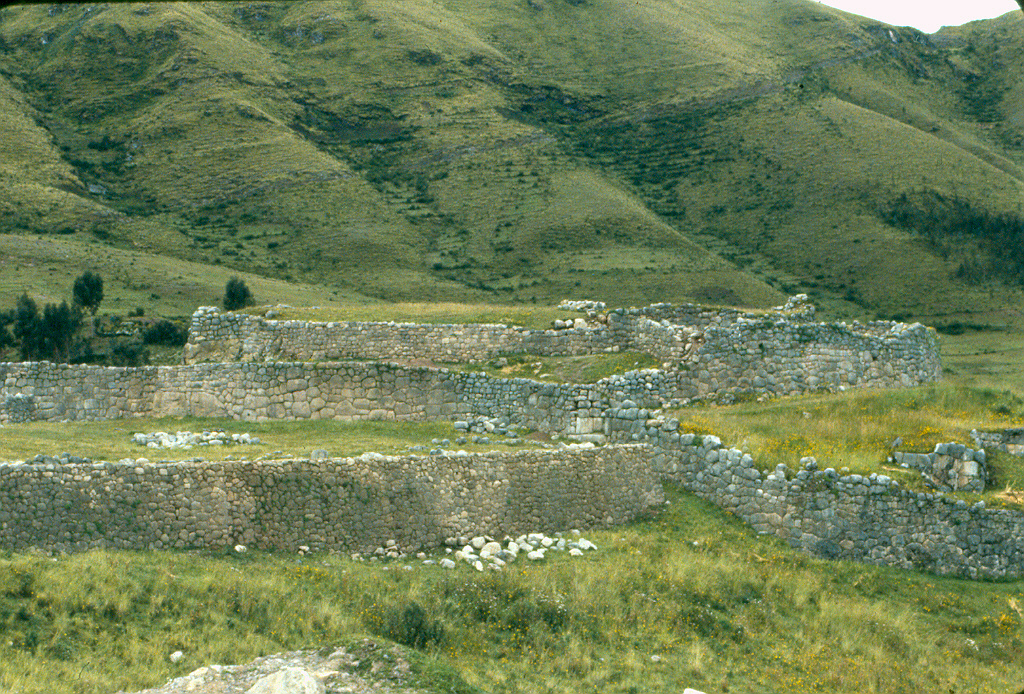This daytime photograph showcases a historic, mountainous region dominated by the ruins of an ancient stone wall that is approximately two to three thousand years old. The scene features a crumbling wall system made of grey and white stones, intertwined with patches of light green grass and natural weeds, including some white flowers. 

The wall remnants outline a site that might have once supported a thriving civilization. Although the structure now stands at a mere five feet in height and is partly destroyed, the stones are still arranged in somewhat square formations, giving a hint of what used to be a more extensive foundation. The wall winds in an irregular path reminiscent of an old castle boundary and displays the ravages of time, with stones fallen to the sides and scattered across the grass.

Surrounding these ruins, the landscape transitions into greener grass as it stretches up into picturesque, rolling hills that ascend into the background, painting a serene tableau of natural beauty framed by the distant mountains. The upper right corner of the image reveals a partial, clear sky, hinting at the expansive, open-air environment of this ancient, yet enduringly beautiful location.